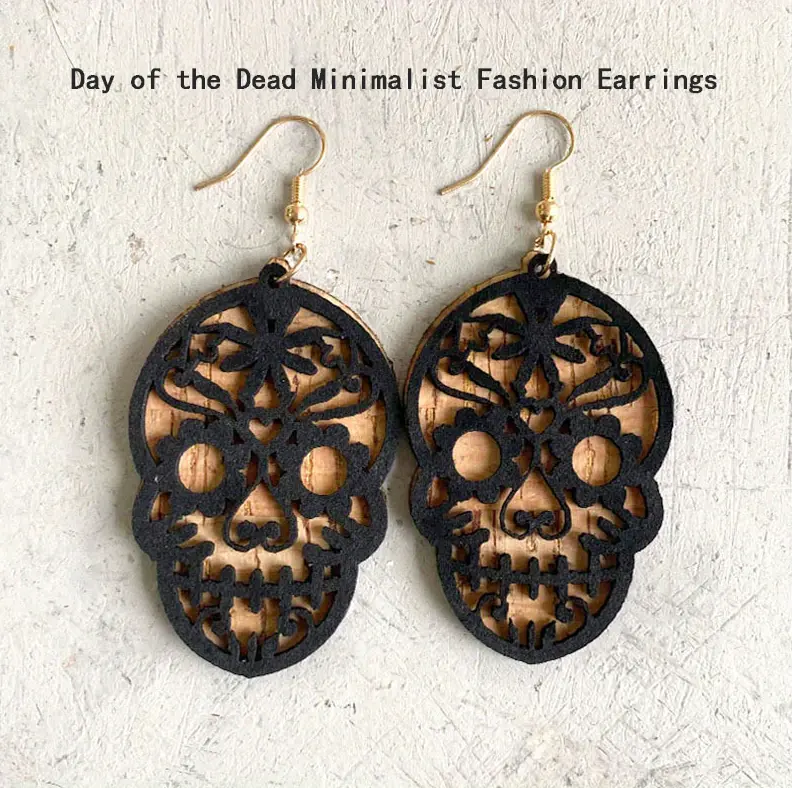The image features a pair of Day of the Dead Minimalist Fashion Earrings. Each earring is adorned with a black skeleton head, showcasing large round eye sockets and distinct nose cavities. They are mirror images of each other, designed to match perfectly when worn as a pair. The earrings are suspended from gold hooks, which are both oriented in the same direction. These features are set against a textured, bone-colored background with a wooden outline and displayed on a square, concrete surface with numerous grooves and carvings. Among the design details, the white background prominently highlights the text "Day of the Dead Minimalist Fashion Earrings" in black letters on the upper part of the image, emphasizing their themed aesthetic suitable for occasions like Halloween.